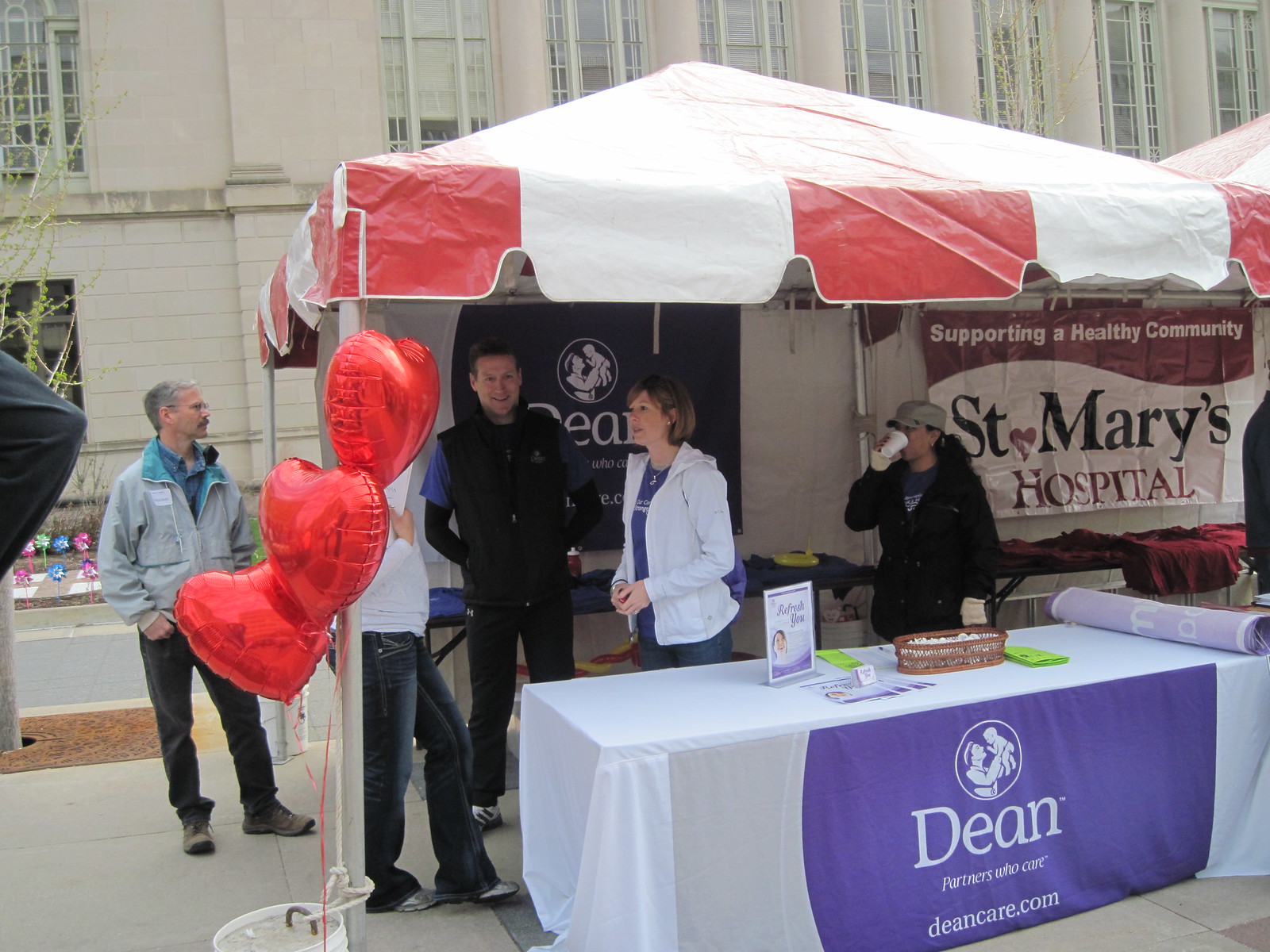This photograph captures an outdoor scene featuring a tent set up with a booth. Inside the tent, there is a table draped with a cloth bearing the text "Dean, Partners Who Care, DeanCare.com." On the table, products, a basket, a sign, and informational papers are neatly arranged. The tent features several red heart-shaped balloons attached to a pole at the front.

The tent is populated by four individuals: three women and one man, who are either standing or sitting and engaging in conversation. The people are dressed for mildly cold weather; one man wears a vest, while one woman sports a white jacket and another a black jacket.

Adjacent to this setup, a sign for "Supporting a Healthy Community, St. Mary's Hospital" is visible, indicating the neighboring booth. Backgrounding the scene is a large building with cream-colored walls and multiple expansive windows, providing a grand backdrop to the friendly and inviting atmosphere of the tent.